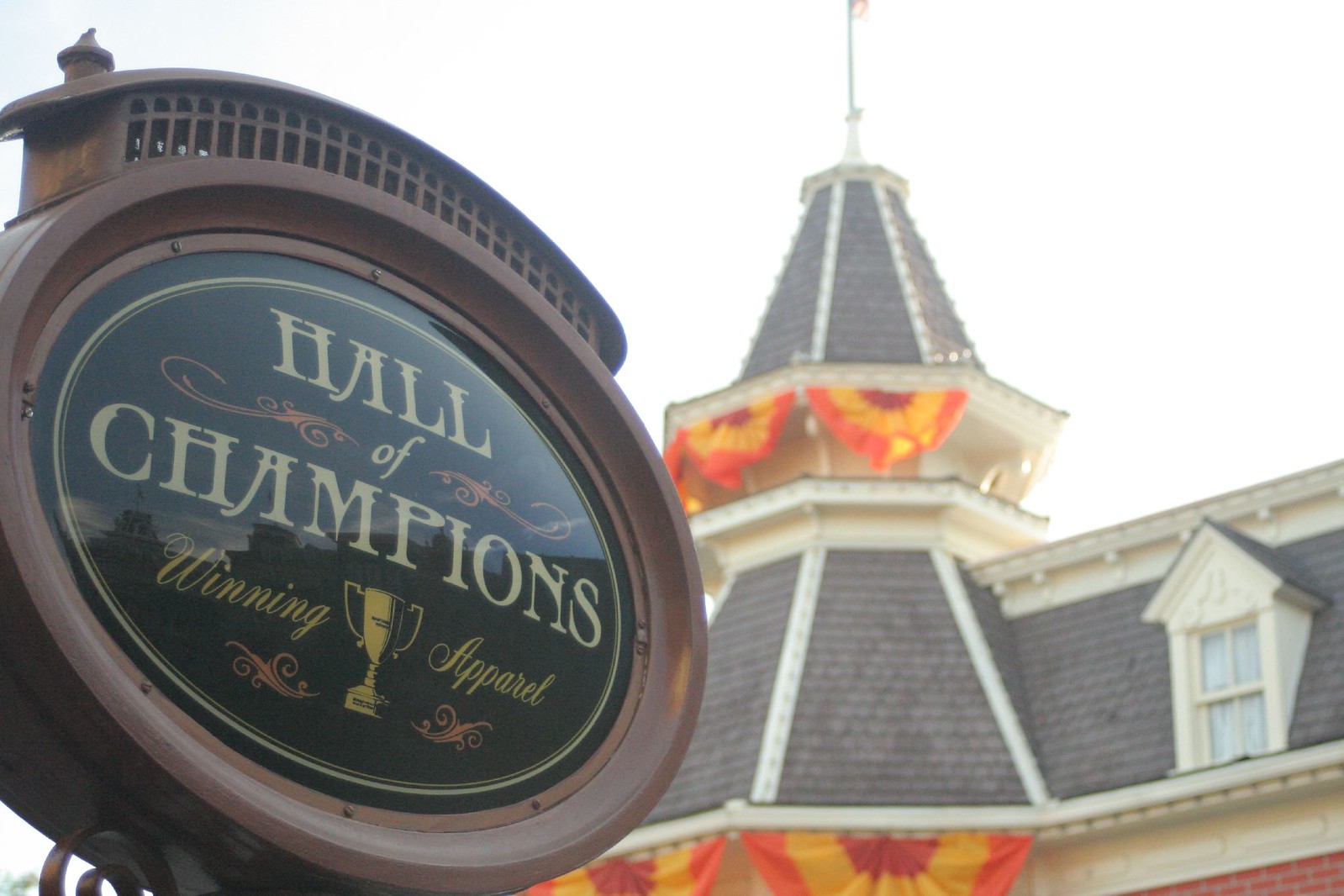The image captures the exterior of a building set against a very white sky, showcasing an old-style, ornately decorated wooden shingle roof. This roof, with its grayish tiles, features a secondary level tower shaped either hexagonally or octagonally, and adorned with a lot of ornate white trim. Draped along the roof's ledges are red, yellow, and orange half-round banners that add vivid accents. Dominating the left side of the image is a prominent round metal sign, set at an angle to the roof. This thick sign, with a glossy black oval center, displays elegant, vintage-style text reading "Hall of Champions, Winning Apparel." Between "Winning" and "Apparel," a yellow trophy is prominently featured, surrounded by decorative images that contribute to its ornate appearance. The intricate details and the combination of text and decorative elements draw attention, creating a visually compelling scene.